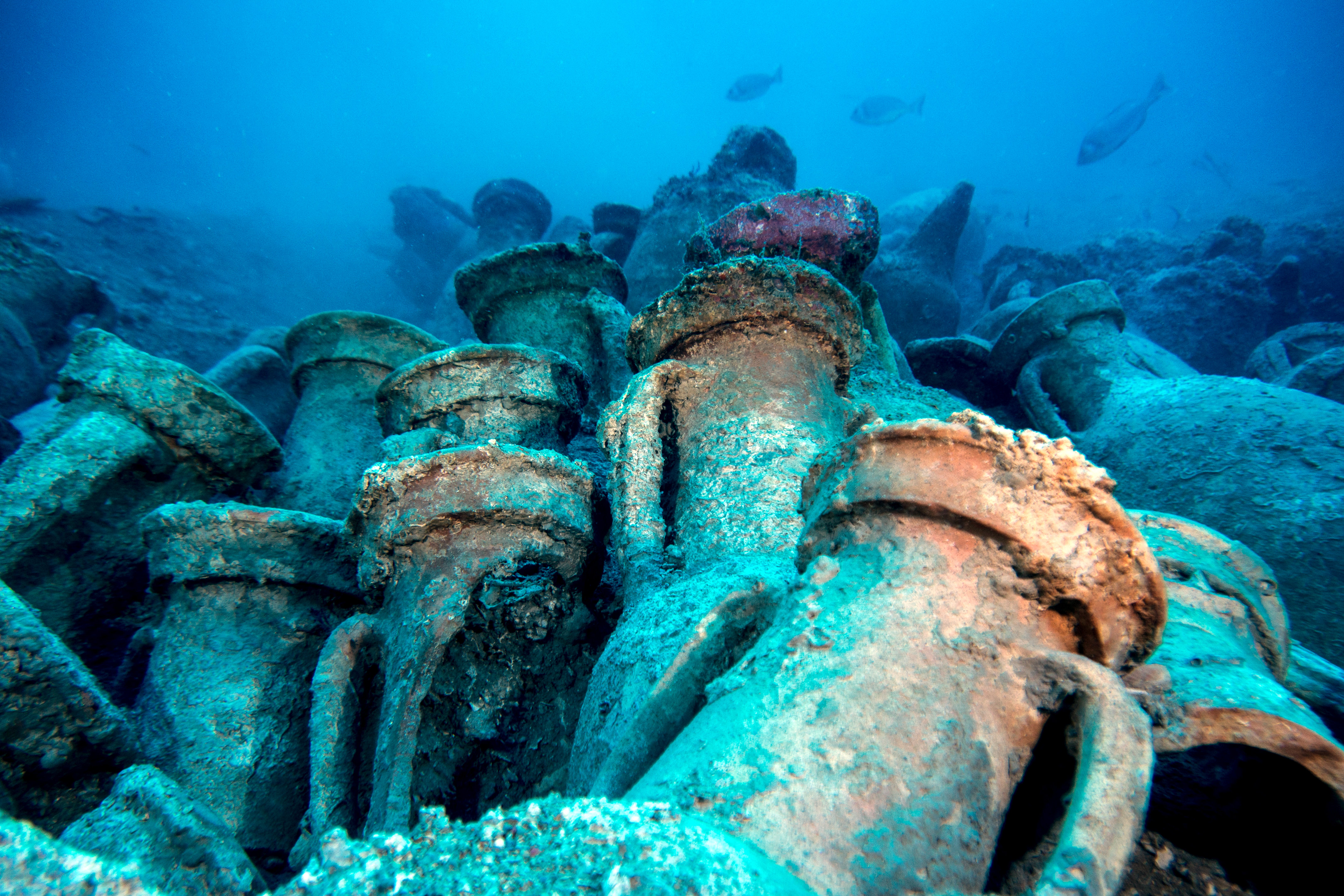This underwater image reveals a large pile of ancient, ornate pots that have seemingly been submerged for centuries. The pots, which are primarily a brownish-red color, are heavily encrusted with rust and barnacles that have taken on aquamarine and turquoise hues. The surrounding water is a deep blue, characteristic of the Caribbean. Some pots are intact while others are broken, displaying their interiors. They are scattered across a sandy ocean floor, accompanied by sea debris and rubble that appears to include more pots. In the background, out-of-focus fish can be seen swimming, adding to the sense of underwater antiquity. The scene shows a captivating blend of natural and historical artifacts, with the textures and colors of the sediment adding to the overall visual intrigue.